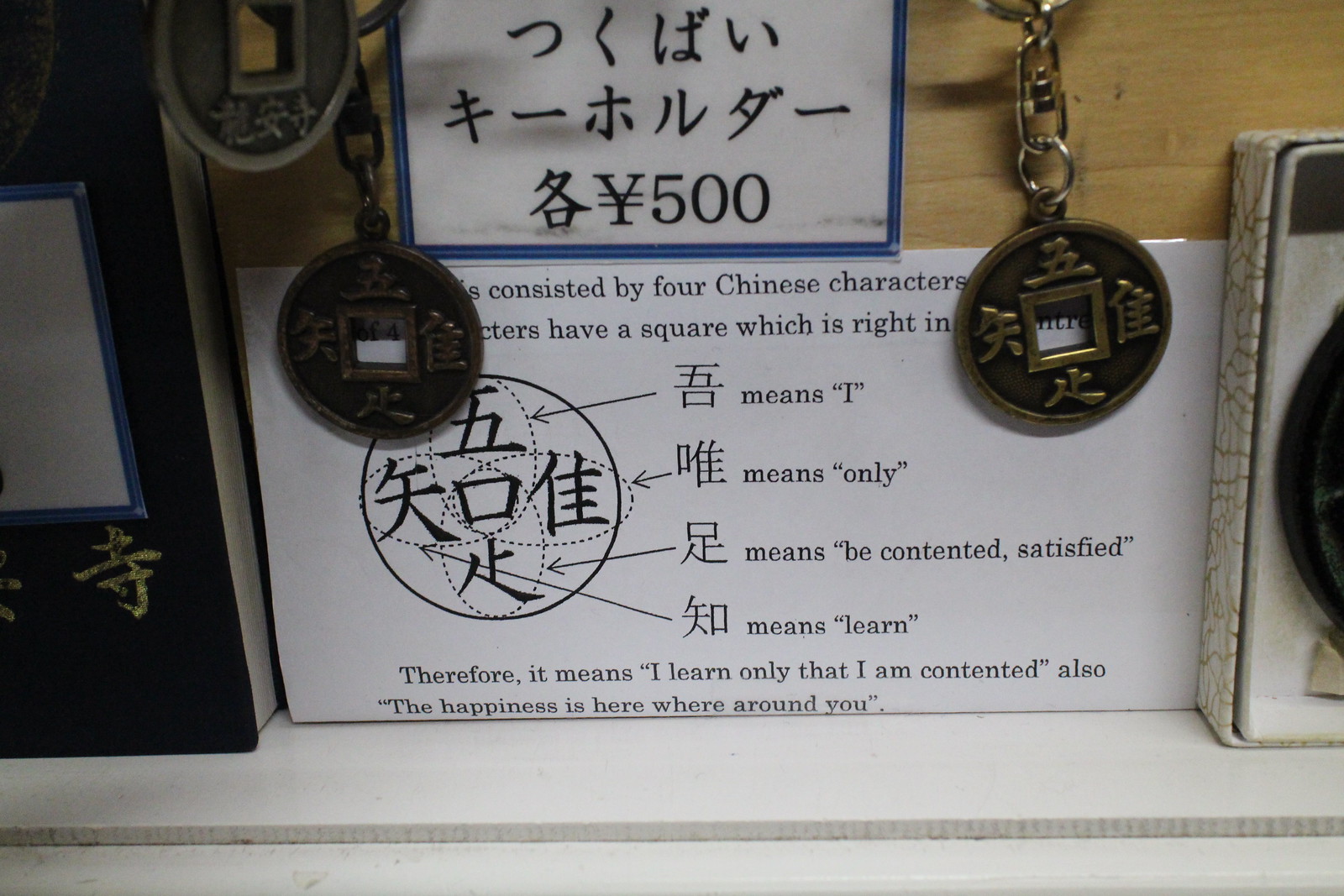This image captures a well-organized display of various accolades and educational materials set against a wooden backdrop. In the center, a wide white paper sign, leaning against the wooden wall, explains the meanings of several Chinese characters in English. Specific translations include "I," "only," "be content," and "learn." Flanking this centerpiece are two medals, each featuring more symbols and a square cutout in the middle, reinforcing the theme of cultural and educational exchange. Above the main sign, a blue laminated piece of paper with Japanese lettering reads "500 yen," indicating a foreign currency value. On the left side of the sign, there's a plaque or book with a dark cover adorned with gold Chinese lettering, adding a touch of authenticity and depth to the scene. The lower edge of the image reveals a white wooden shelf, further grounding the display in a tangible setting. This image likely represents an educational setting, perhaps a school, where recognition and learning about different cultures are prominently featured.